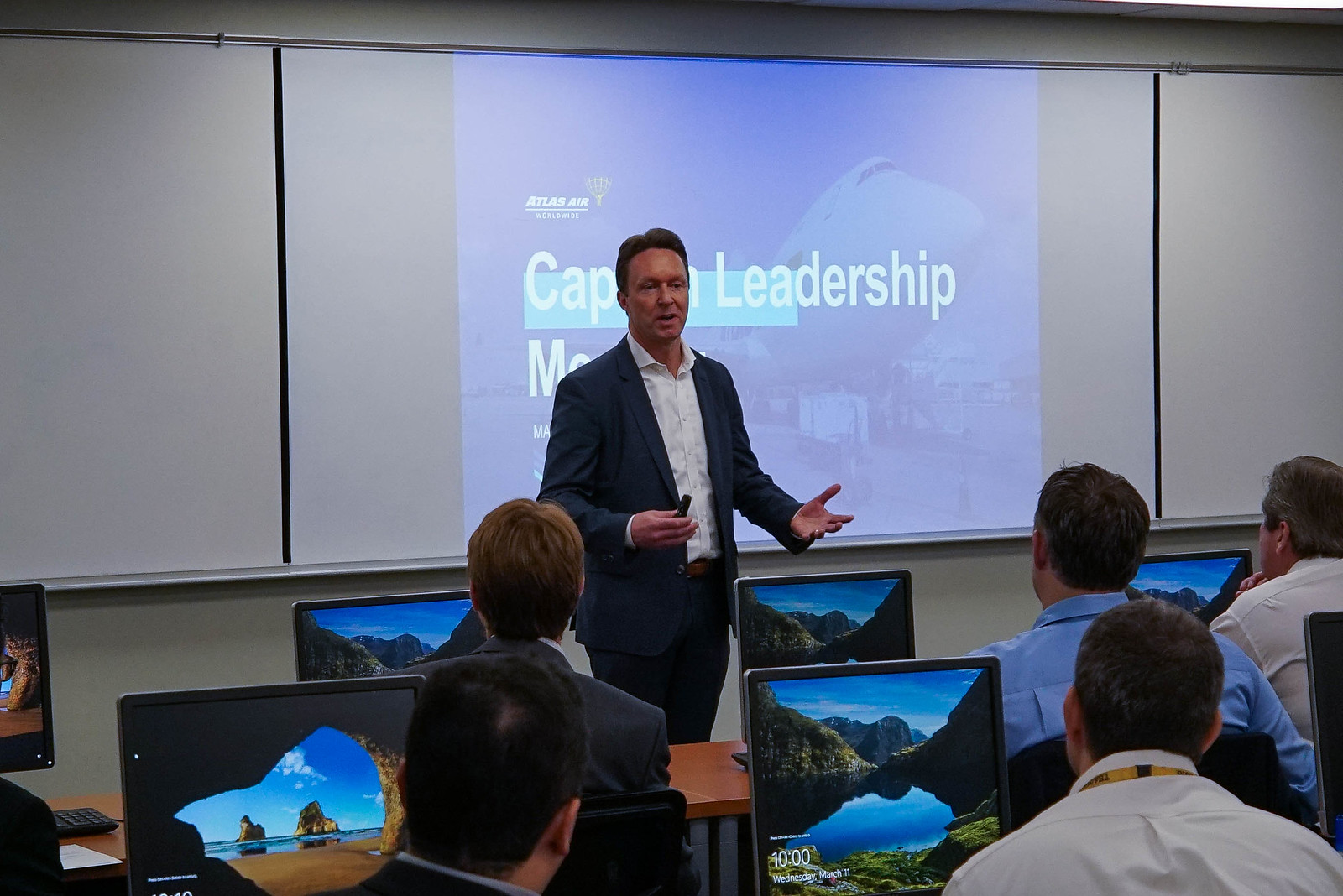This photograph captures a mid-aged, white male presenter with short dark brown hair, standing at the front of an office or conference room. The man, dressed in a dark blue suit and white dress shirt, gestures with his right hand while holding what appears to be a clicker. Behind him, a three-panel whiteboard displays partial text including the word "leadership" along with an image, possibly of a building. In front of the presenter, a diverse audience of men, seen from the back, are seated with laptops open. These laptops show varying screen contents, with most displaying a scene featuring mountains and a lake, while one on the left side shows an image of two rocks and an ocean. The setting suggests a professional or educational conference, emphasizing leadership, where the attendees are engaged and following along with the presentation.